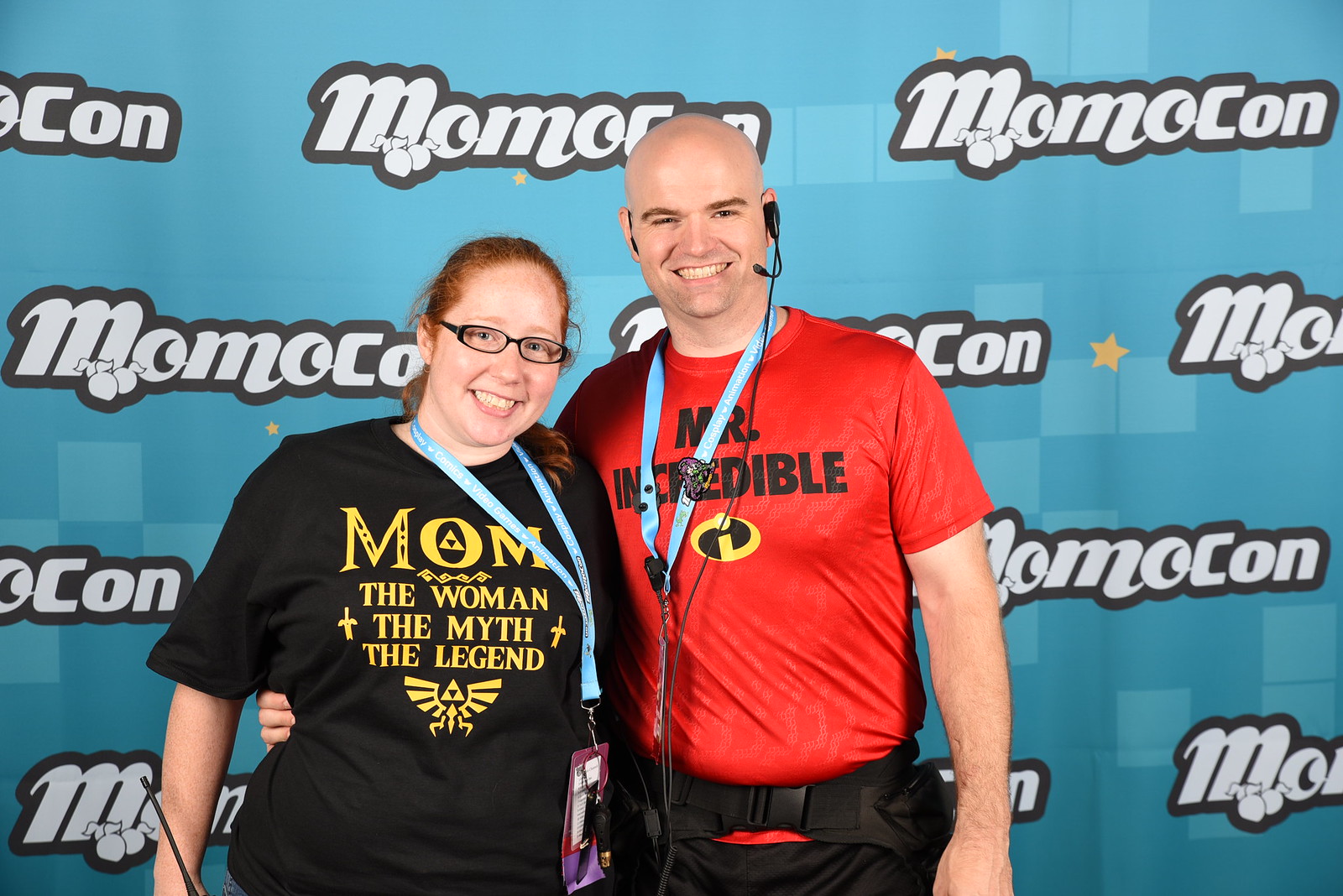This photograph captures two people standing against a mostly blue wall adorned with the logo "Momocon" repeatedly written in white letters outlined in black, accompanied by yellow stars. The woman on the left has reddish-brown hair pulled back into a ponytail and is wearing black-framed glasses. She's smiling and dressed in a black t-shirt that reads "M.O.M.O. The woman, the myth, the legend," with a bird graphic below. She also has a lanyard with items hanging from it. The man on the right has a bald or shaved head, is smiling, and sports a red t-shirt with "Mr. Incredible" printed on it, along with a corresponding logo. He wears a blue lanyard, dark pants, and a headset over his ears. Additionally, he's wearing a fanny pack and has his arm around the woman's waist.